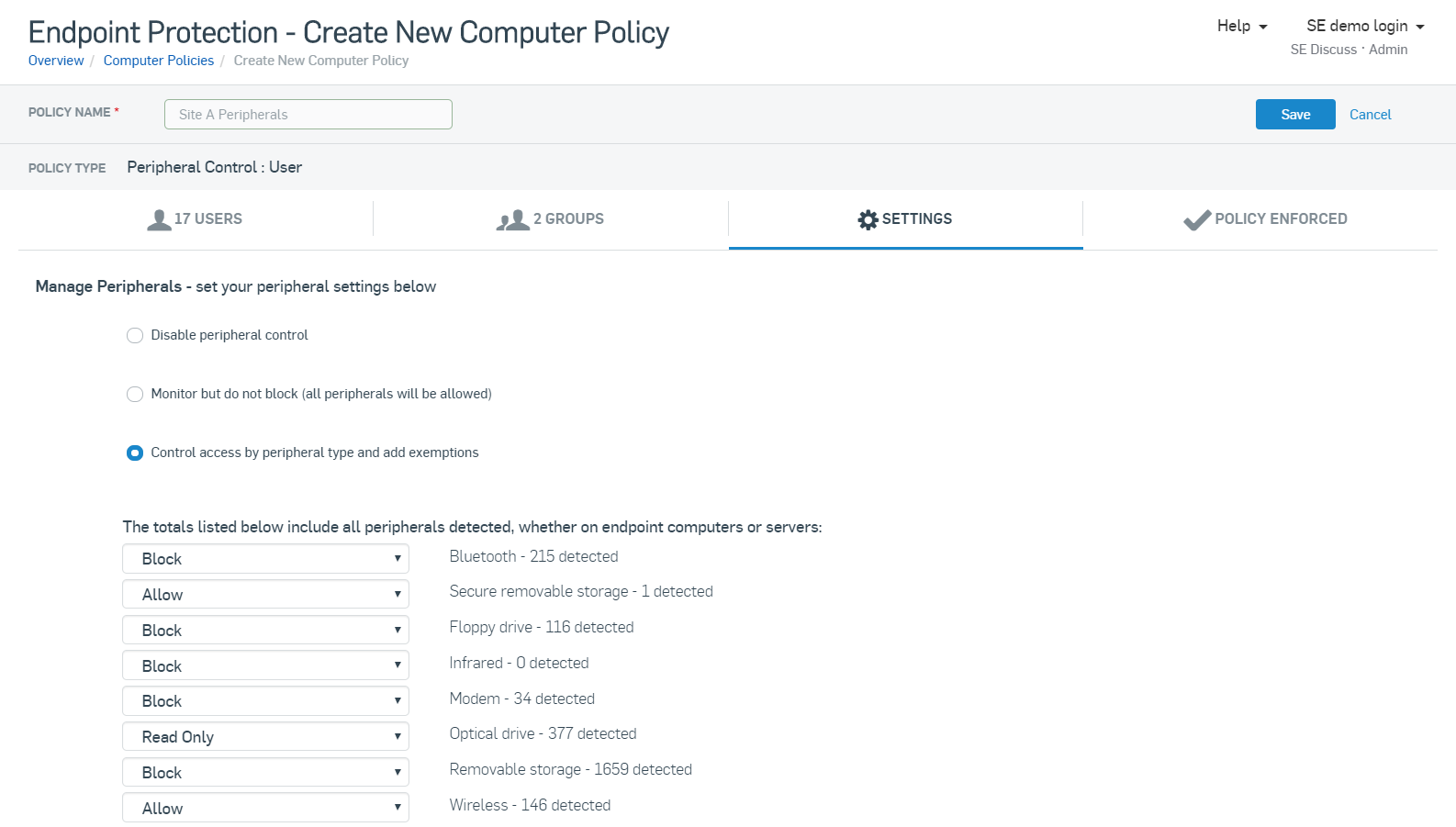The image is a screenshot of a computer interface for creating a new policy in an endpoint protection system. 

At the top, the header section is white with two sections of text on either side. On the left, in black text, it reads "Endpoint Protection - Create New Computer Policy". On the right side, in black text, it says "Help SE Demo Login", and below that in gray text, it says "SE Discuss and Admin".

On the left-hand side, in a vertical blue menu, it reads "Overview / Computer Policies" with each section separated by a gray slash. The "Computer Policies" section is highlighted in blue. Below this, in gray text, it reads "Create New Computer Policy".

The main section of the interface is a large gray rectangle. At the top, in black text, it says "Policy Name" marked with a red asterisk indicating a required field. There is an outlined input box below that, filled with the text "Site A Peripherals".

On the right side, there are blue buttons: one for "Save" (with white text) and another for "Cancel". A thin gray line separates these from the next section.

Below this line, it says "Policy Type" followed by "Peripherals Control.User" in black text. The background remains white, and underneath this is a vertical gray line dividing sections for "Users" and "Groups".

In bold black text, it says "Settings", accompanied by a black gear icon and underlined in blue. Adjacent, it states "Policy Enforced". Underneath, in black text, it reads "Manage peripherals: Set peripheral settings below. Disable peripheral control mindset but do not block all personnel will be shown."

Next to this text are several options presented as circles. One of these circles is blue, indicating it is selected, with the option "Control Access by Peripheral Type". The interface invites further action with a prompt to "Add Example."